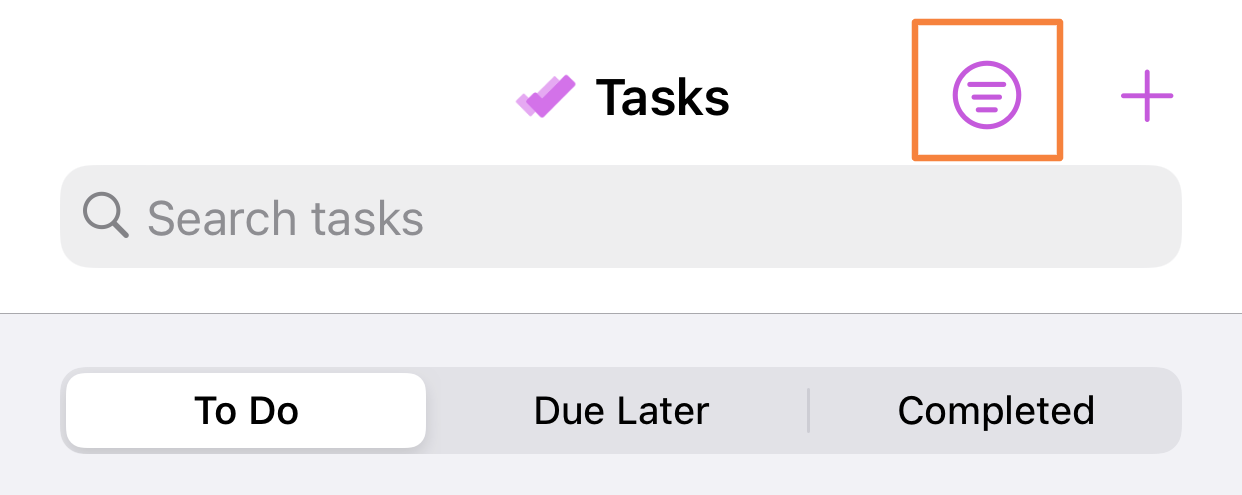This image is a simple, rectangular task management interface with a minimalist design. It features a partially white and partially light gray background, and is significantly wider than it is tall.

At the top center of the image, "Tasks" is displayed in bold black text against a white backdrop. To the left of this text, two overlapping purple check marks are depicted, with the darker purple check mark partially covering the lighter one. To the right of the word "Tasks," there is a white box with a red border. Inside this box, a purple circle contains three horizontal purple lines of descending width, and a purple plus sign is positioned in the top right corner of the box.

Below this, a gray text bar includes a magnifying glass icon on the left side and the words "Search Tasks" within the bar, indicating a search function.

Further down, a gray rectangle hosts three tabs for task categorization. The first tab, labeled "To Do," is highlighted with a white background and black text. The second and third tabs, labeled "Do Later" and "Completed," respectively, have gray backgrounds with black text. This structured layout suggests an organized approach to managing tasks.